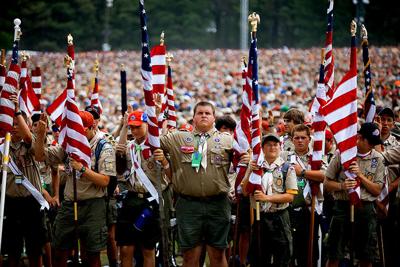The image depicts a group of what appears to be Boy Scouts or soldiers, all of whom are Caucasian men, holding the American flag with noticeable pride and seriousness. Dressed in traditional khaki tops and shorts, some of the young men display patches and medals on their shirts. The American flag, featuring red and white stripes along with a navy blue section adorned with stars, is prominently visible. The scene takes place outdoors, with a large crowd gathered, suggesting a significant event or ceremony. The background reveals an expanse of greenery, further emphasizing the well-attended nature of the gathering.